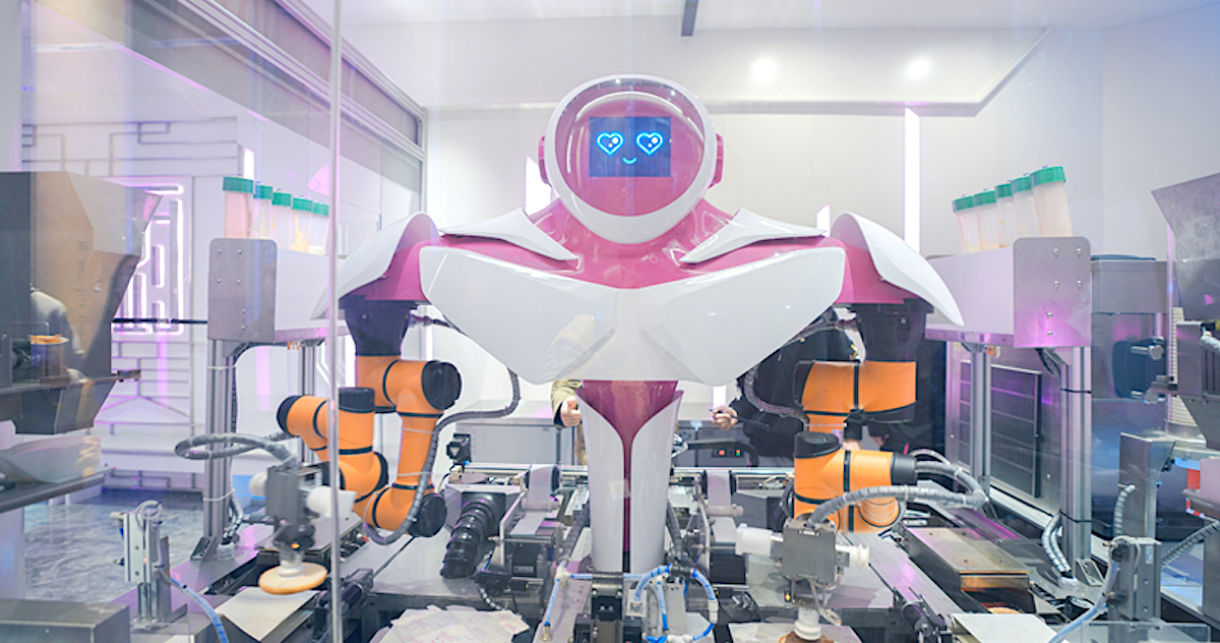The image captures a humanoid robot positioned centrally in a laboratory or factory display area, behind a protective panel of glass. The robot itself is composed predominantly of white structures with accents of red and pink. Its upper body showcases wide shoulders, and the lower part tapers into a tubular design blending white and pink elements. The robot’s head has a dark blue face with a pink hue and displays an expressive, happy demeanor through light blue heart-shaped eyes and a squiggly line representing a mouth.

On either side of the robot, there are distinct yellow camera-like fixtures, possibly part of the lab's monitoring equipment. The background is mainly white, featuring silver machinery, some which might mimic a restaurant setup, including items that resemble stoves and various machine parts indicative of an assembly or testing lab left and right. The setting also includes visible white ceilings, reinforcing the clean, structured environment of the lab.